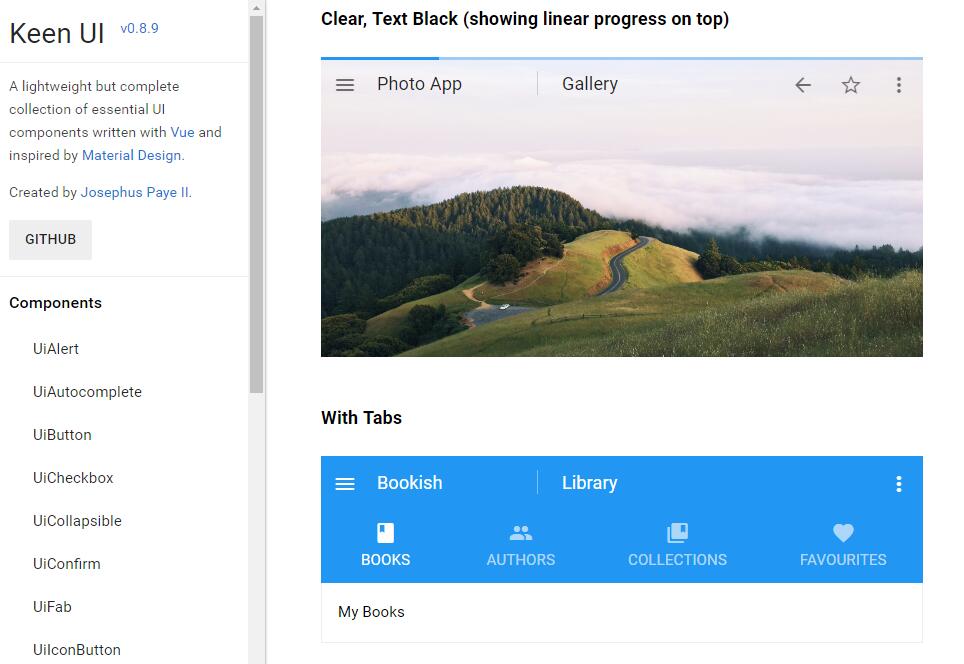**Descriptive Caption:**

The image is a detailed screenshot of a rectangular landscape-oriented interface, likely taken from a monitor or laptop. The screenshot is divided into two primary sections with a white background and no borders. 

**Left Panel:**
- Occupies about 30% of the image.
- Contains controls and instructions delineated by a vertical scroll bar on the right side.
- The scroll bar has a top half in dark gray and a bottom half in light gray, indicating scrolling.
- At the very top of the scroll bar, there’s an upward-facing arrowhead.

**Top Section of the Left Panel:**
- The panel starts with the text "Keen UI" in the largest font, aligned in the upper left corner.
- To the right of "Keen UI", it displays "V 0.8.9" in a smaller font.
- Below this is a horizontal underline, followed by a text description: "A lightweight but complete collection of essential UI components written with VUE and inspired by Material Design." The words "VUE" and "Material Design" are in all caps and colored blue, likely hyperlinks.
- Beneath this, there's a space followed by "Created by Josephus Paye II," also in blue.

**Middle Section of the Left Panel:**
- Features a gray box with the text "GITHUB" in dark font, all caps.
- Another horizontal line runs across the panel below the GitHub box.

**Bottom Section of the Left Panel:**
- Contains a header labeled "Components" in bold, left-justified.
- Below the header are eight indented component names listed vertically: 
  - UI Alert
  - UI Autocomplete
  - UI Button
  - UI Checkbox
  - UI Collapsible
  - UI Confirm
  - UI Fab
  - UI Icon Button
  - Each component name follows a specific capitalization pattern with the "U" capitalized, "I" lowercase, and the next letter capitalized.

**Right Panel:**
- Occupies the remainder of the image, separated from the left panel by the vertical scroll bar.

**Top Section of the Right Panel:**
- Displays "clear" in bold, black text, left-justified, followed by "(showing linear progress)" in parentheses.
- Below this text is a landscape photograph featuring a hilly, tree-laden area with grassy foreground, a curving central road, and a cloudy sky stretching into a lighter blue. No people or sun are visible.

**Header Above the Landscape Photograph:**
- Contains: 
  - Left: Three horizontal bars (menu icon) and "photo app".
  - Center: "gallery".
  - Right: Three icons—a leftward-pointing squat arrow, an empty star, and three vertical dots—all in gray text.

**Bottom Section Below the Landscape Photograph:**
- Features a left-justified, bold header "with tabs".
- Beneath the header is a medium to light blue horizontal rectangle with white text.
  - Top Row: 
    - Left: Three horizontal bars (menu icon).
    - Middle: "bookish".
    - Center: "library".
    - Right: Three vertical white dots.

**Middle Section of the Blue Box:**
- Contains four sections, each with an icon above a word:
  - "BOOKS" with a portrait rectangle icon.
  - "AUTHORS" with overlapping head and shoulders icons.
  - "COLLECTIONS" with overlapping squares/paper icons.
  - "FAVOURITES" (British spelling) with a heart icon.
- The “BOOKS” section appears highlighted, glowing brighter than the others.

**Bottom Section of the Blue Box:**
- Displays the text "my books" in smaller, left-justified text.

This screenshot depicts what appears to be a photo editing or management interface with a focus on user interface component listings on the left and a gallery view on the right.